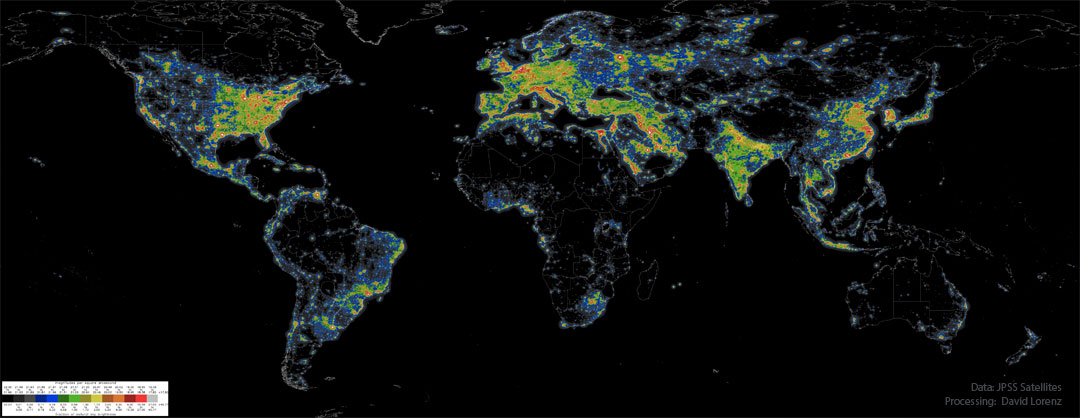In this detailed map, the entire world is depicted on a black background, providing a striking contrast to the colorful data presented. Located in the lower-left corner is a legend, a white strip illustrating a spectrum of colors starting from black and gray, progressing through shades of dark blue, light blue, dark green, light green, and lighter green, and culminating in yellow and various shades of red. 

The color scheme is used to differentiate areas on the map. The United States displays a significant amount of blue and orange hues on the western half, transitioning into areas of blue and green in the central states, with the eastern part predominantly showing green and red.

In South America, the coastal regions feature some blue, particularly on the east side where blue and yellow dominate. The map reveals that Europe is covered in a mix of yellow, green, and blue, signifying a blend of traits or data points. Meanwhile, Africa shows limited but notable regions of blue and yellow concentrated at the southern tip. 

This colorful representation across continents provides a visually rich and informative overview of the varying data points mapped across the world.